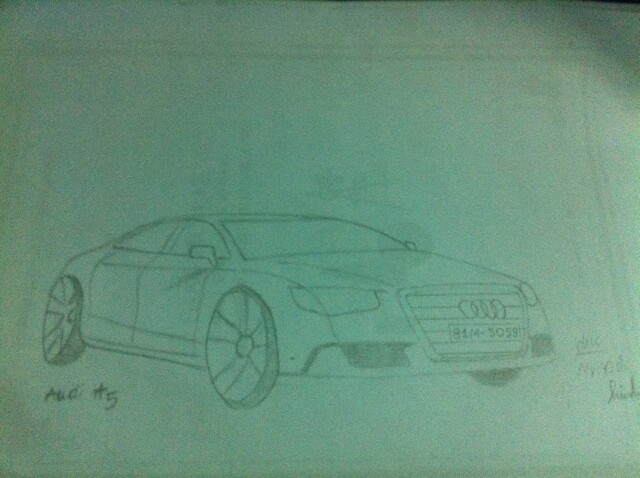This is a detailed hand-drawn illustration of a sedan, possibly an Audi A5, rendered on standard printer paper. The car is depicted in a light mint green hue, though the lighting might be influencing this perception, intensifying towards the center of the page. The drawing appears to be done on the reverse side of a flyer or similar printed material, as faint black outlines are visible through the paper. The bottom left corner features a somewhat unclear inscription, likely identifying the car model as an Audi A5. The right side of the drawing includes what seems to be the artist's signature, adding a personal touch to the artwork.